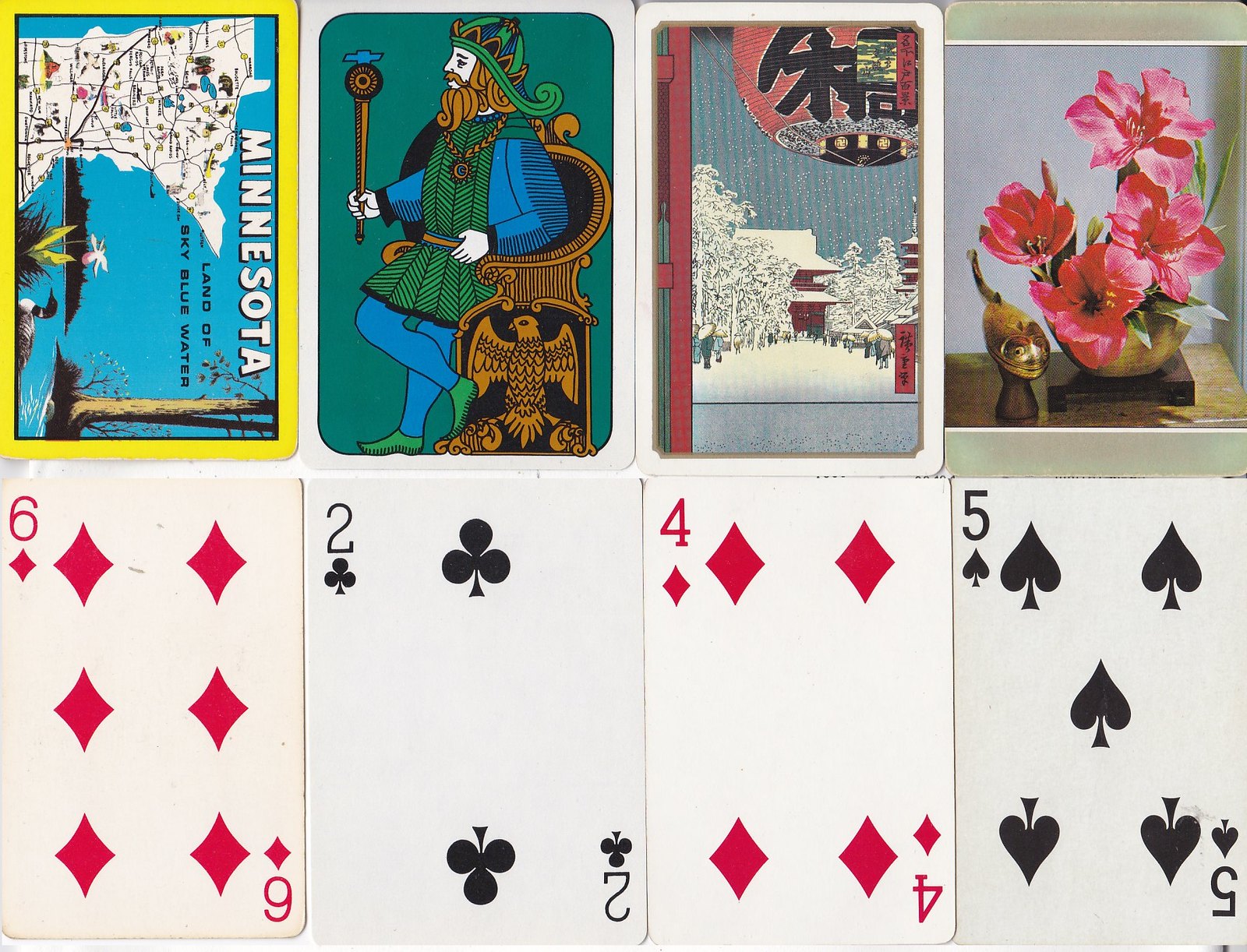The image features eight playing cards, with four cards face-up and four cards face-down. The face-up cards consist of a 2 of Clubs (black), a 4 of Diamonds (red), a 6 of Diamonds (red), and a 5 of Spades (black). The face-down cards display a variety of designs on their backs. One card back has a detailed map of Minnesota, known as the Land of 10,000 Lakes, depicted in sky blue water colors. Another card features a Chevy emblem held by what appears to be a figure, possibly a joker, jack, or king, seated on a chair adorned with an eagle on the side; and the background is a vibrant green. The third card illustrates a snowy Japanese landscape, complete with snow-covered white trees, a red paper mache ball with a Japanese letter in the foreground, and a red building set against a gray sky in the background. The fourth card shows an arrangement of flowers with a small wooden kitty figurine on a wooden stand, set within a room.